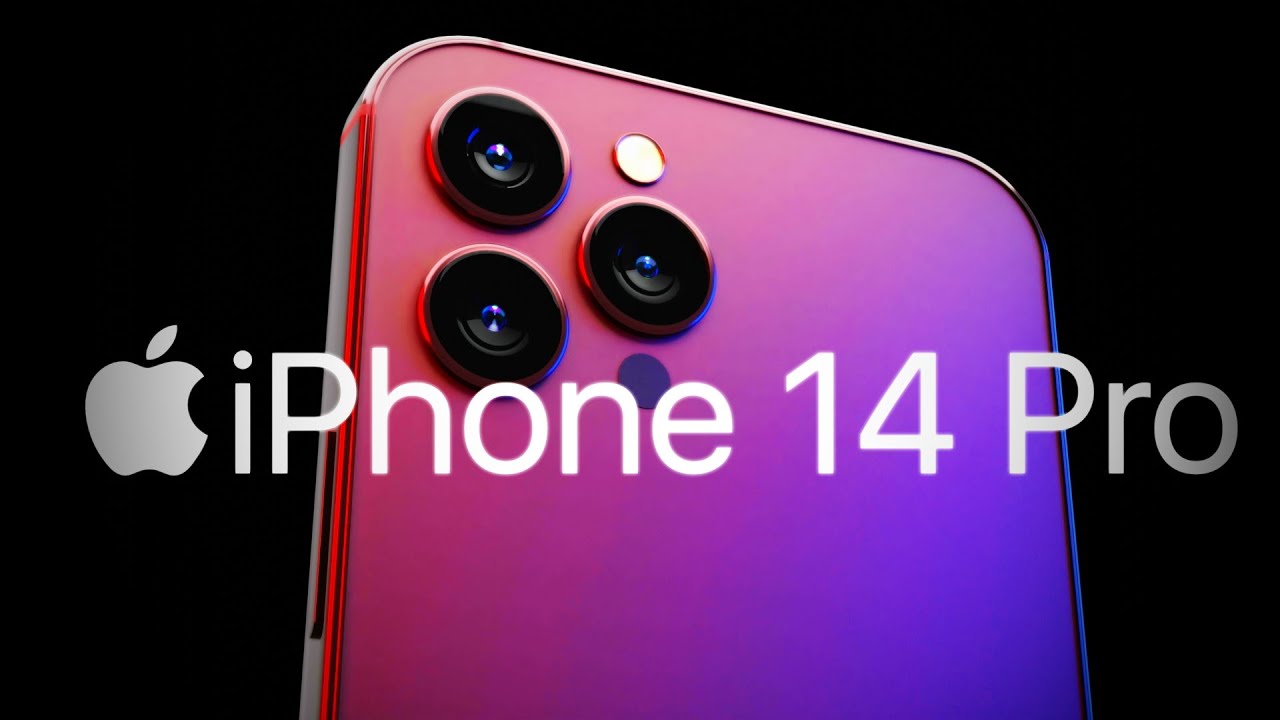A high-quality, professional banner for the iPhone 14 Pro is showcased, captured as a meticulous screenshot. The visual centerpiece is a glossy photograph, focusing on the top corner of the iPhone 14 Pro. Displayed at an angle, the image prominently features the phone's edge on the left-hand side, accentuating its sleek design.

Three round, sophisticated cameras are highlighted in the top left-hand corner on the back of the phone. These cameras are arranged in a triangular formation, with one at the top left corner, another directly below it, and the third positioned slightly off-center to the right of the other two.

Adding to the allure, the banner is illuminated with a stunning gradient, starting with red on the top sides, transitioning to pink and purple in the middle, and concluding with blue at the bottom right-hand corner, all set against a stark black background. 

The text “iPhone 14 Pro” is displayed prominently across the middle of the banner in Apple's signature sans-serif font, rendered in white but edited to create a fading effect towards both edges, culminating in a faint glow in the center. 

The image also showcases intricate details, such as a small white circle above and a darker circle below the right camera, likely representing additional sensors or flash. The back of the phone, with its glass surface, is subtly indicated by a slight inset from the phone's rim, accentuating its premium construction.